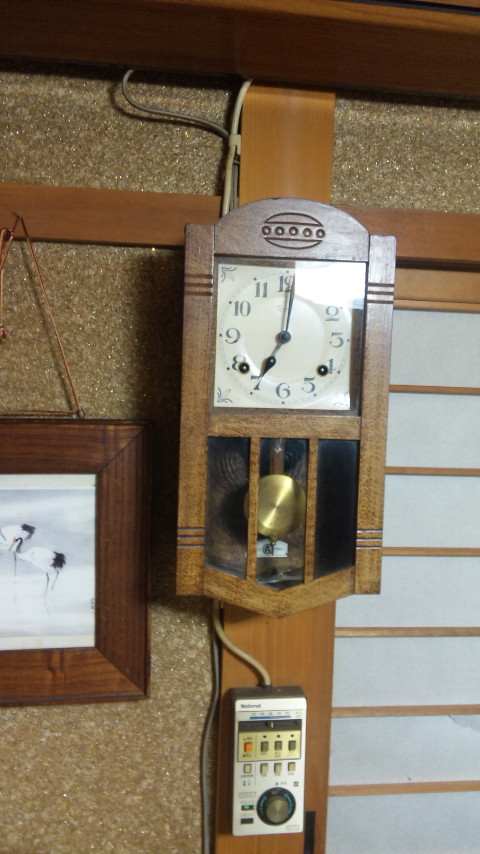The image showcases an intricately designed clock illuminated by a bright flash, making its details stand out vividly. The clock is mounted on a rustic stone wall, which serves as the background. One can observe a series of white squares and rectangles at the bottom right, possibly decorative tiles, with a wooden strip running horizontally across them. On the left side of the image, there is a photo frame containing a picture of a person sitting on a bench, framed in smooth, rounded wood. 

The clock face features all twelve numerical indicators, with the minute hand pointing at 12 and the hour hand at 7. Additional marks are visible on the top left and top right sections of the clock, perhaps as decorative elements. A pine cone, simply hanging down and not in motion, adds to the rustic charm. An electronic device, featuring various buttons and a prominent black dial, is attached to the clock via a cable and is situated in the center of the image. The composition captures a blend of vintage and modern elements, possibly reflecting a cozy, eclectic living space.